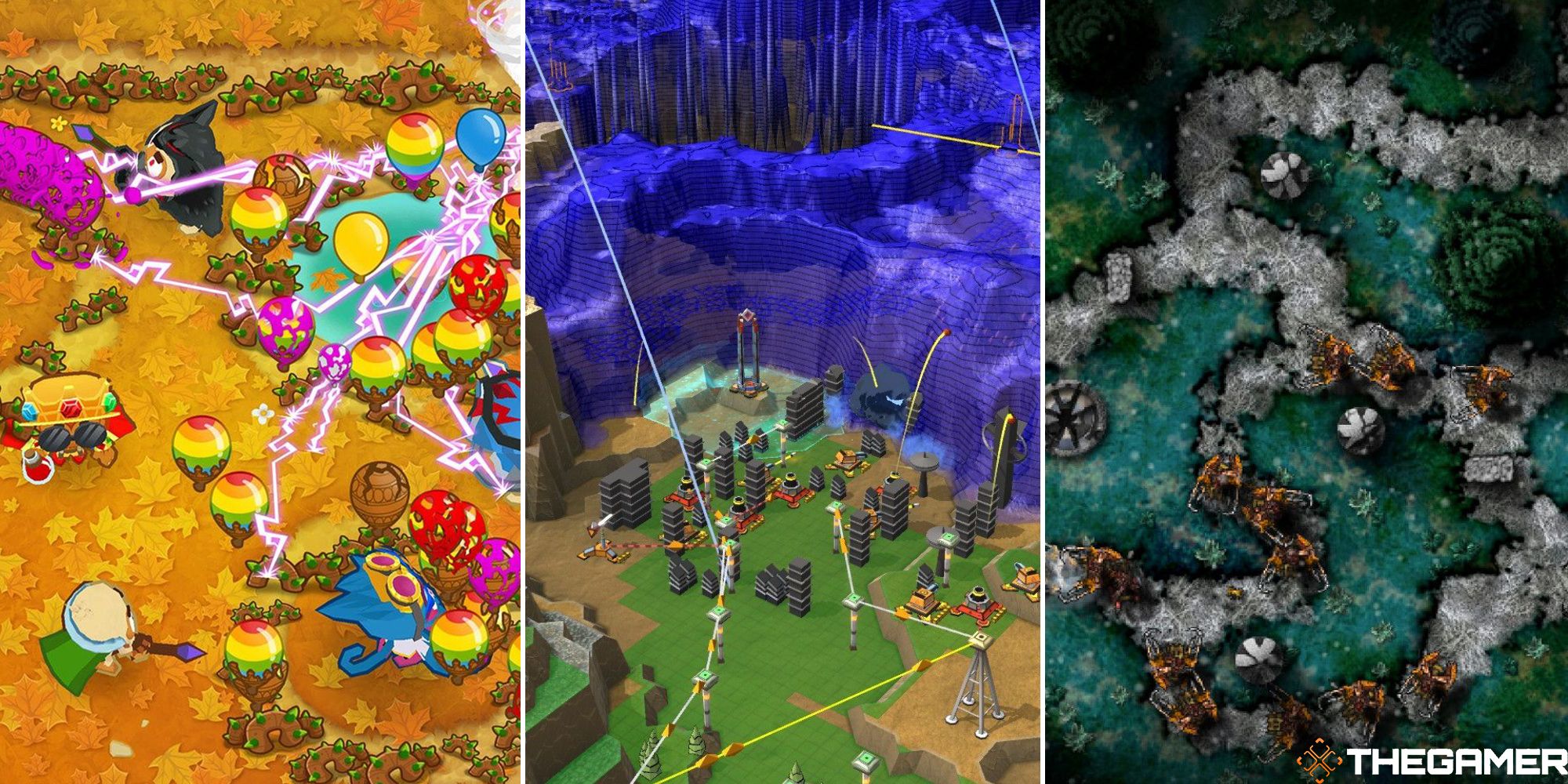The image comprises three side-by-side rectangular panels, each depicting vibrant scenes from different video games. The left panel features an orange-hued ground scattered with autumn leaves and various colorful balloons surrounding a pond. There is a creature, possibly a cat or a dog, emitting electrical rays at the balloons, while a man in a green cape wields a wand topped with a purple stone, sending out pink lightning. The middle panel illustrates a dark, cave-like environment with a blend of blue, purple, and black tones reminiscent of a Minecraft scene. At the bottom, a green and brown area filled with equipment and figures emits light rays between them, creating a dynamic, battle-like atmosphere. The right panel presents a gray pathway interspersed with orange segments, bordered by green terrain. Various wheels and objects are scattered throughout, depicting a maze-like scene. Notably, the bottom right corner of this image contains the text "The Gamer."